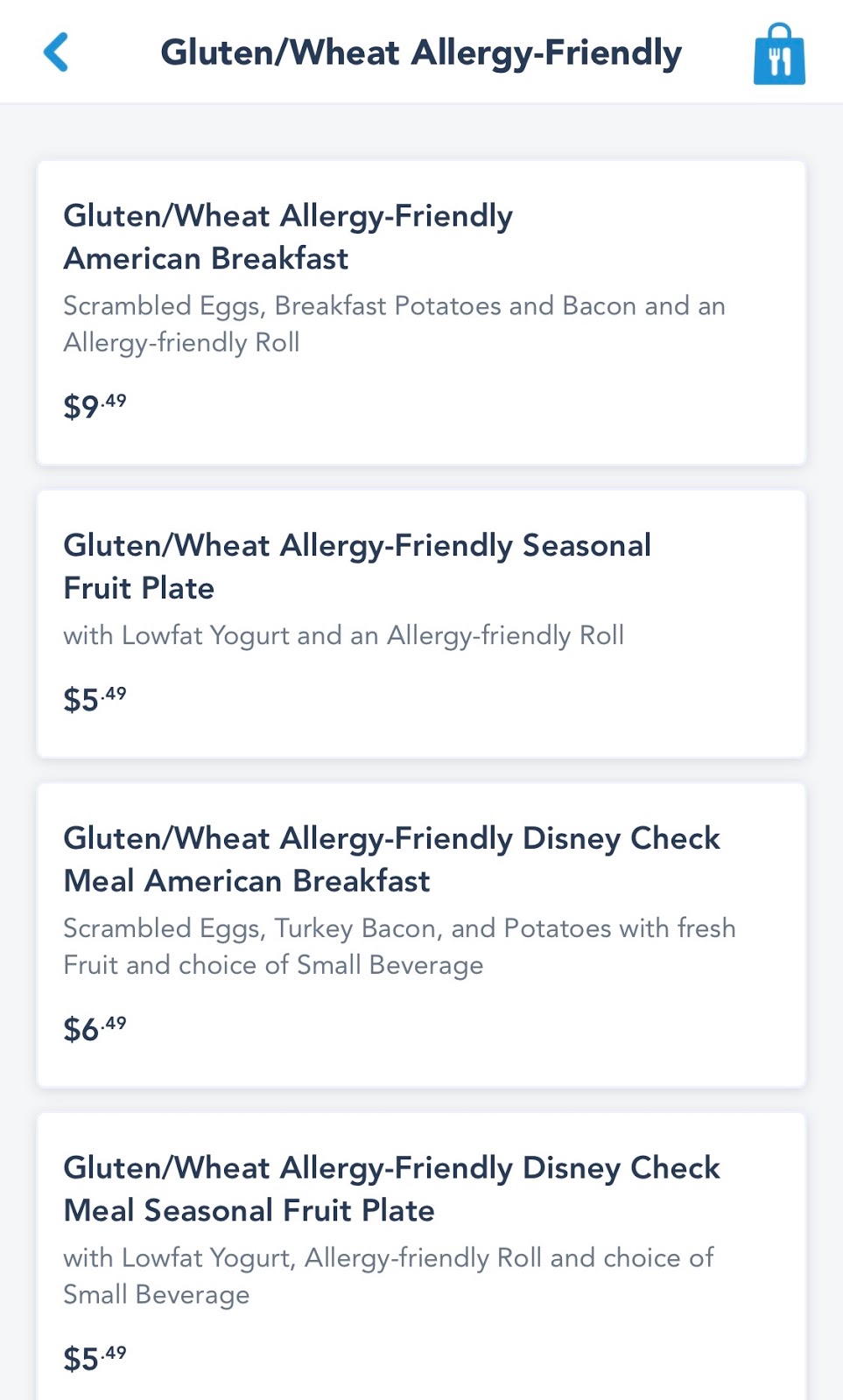The image showcases a menu with options specifically designed to accommodate gluten and wheat allergies. The top section features a label reading "Gluten/Wheat Allergy Friendly," with a blue less-than symbol on the left and a blue bag icon on the right, all set against a gray background. Below this label are four white rectangular boxes, each detailing a different meal option:

1. "Gluten/Wheat Allergy Friendly American Breakfast" - Includes scrambled eggs, breakfast potatoes, bacon, and an allergy-friendly roll, priced at $3.49.
2. "Gluten/Wheat Allergy Friendly Seasonal Fruit Plate" - Features a selection of fresh fruits, low-fat yogurt, and an allergy-friendly roll, priced at $5.49.
3. "Gluten/Wheat Allergy Friendly Disney Check Meal: American Breakfast" - Contains scrambled eggs, turkey bacon, breakfast potatoes, fresh fruit, and a small beverage, priced at $6.49.
4. "Gluten/Wheat Allergy Friendly Disney Check Meal: Seasonal Fruit Plate" - Offers seasonal fruits, low-fat yogurt, an allergy-friendly roll, and a small beverage, priced at $5.69.